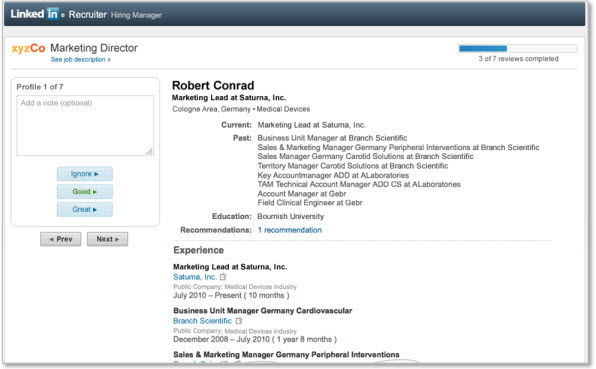The LinkedIn page features a dark gray header, prominently displaying the LinkedIn logo on the left. Just below the header, the terms "Recruiter" and "Hiring Manager" are visible against a white background with a light gray top border. On the top left corner of the main section, there is a green logo with the text "XYZ Code." To its right, the title "Marketing Director" is written in bold black letters. Below this title, a small, blurry blue hyperlink offers options to "Save Job Description" or "See Job Description."

In the upper right corner of the page, a status bar indicates that 3 out of 7 reviews have been completed, with the progress visually represented by a dark blue line partially filling the gray bar, approximately 40% of the way. Underneath the status bar, the name "Robert Conrad" appears in black text, followed by the role "Marketing Lead at Satoma Incorporated" in smaller text. Below this, in slightly smaller and non-bold text, it states "Cologne Area, Germany Medical Devices." Further down, there is a column listing "Current," "Past Education," and "Recommendations."